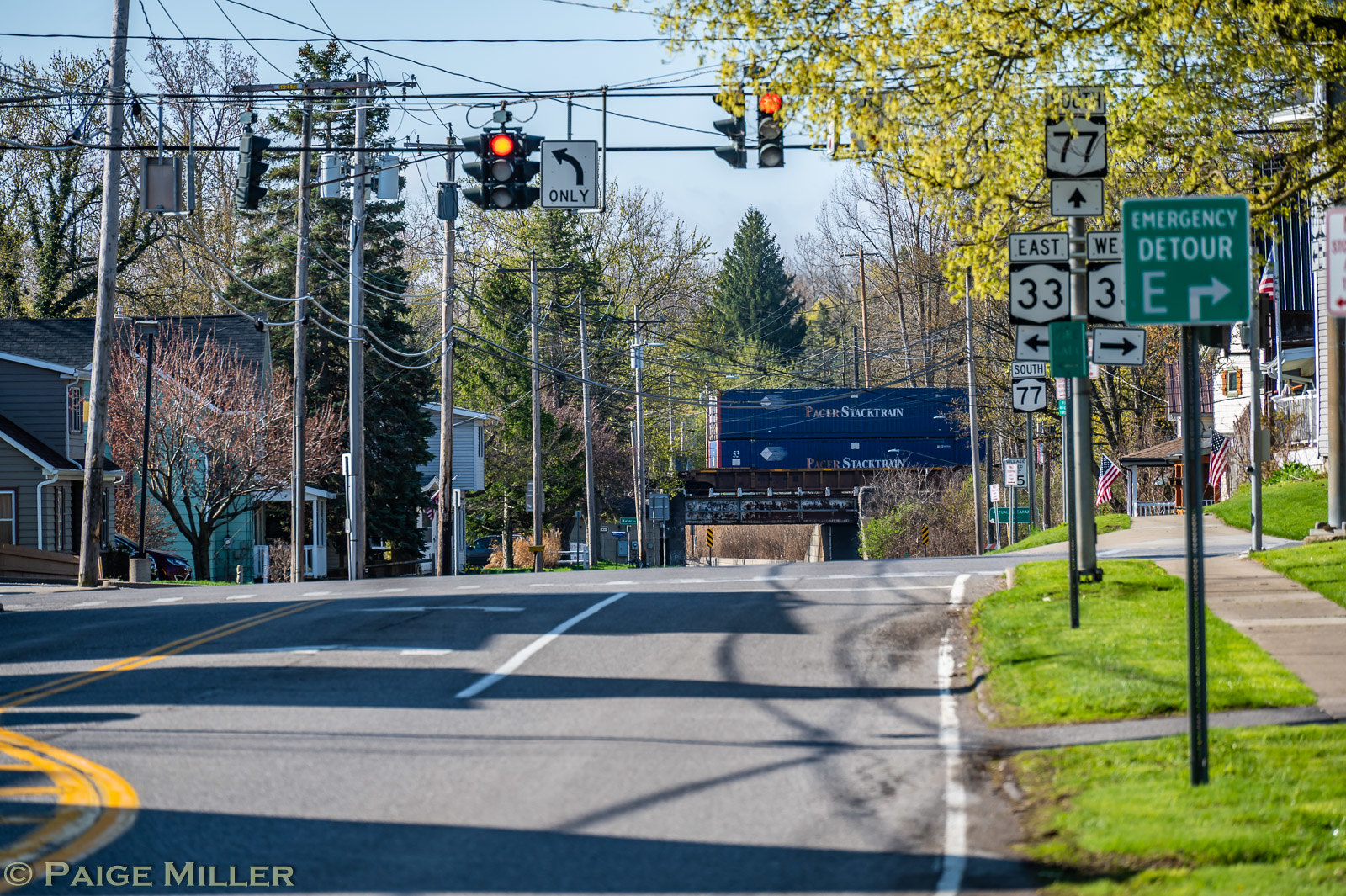The image captures a typical American suburban town intersection during daytime with a clear blue sky. The center of the photo prominently features a set of traffic lights shining red, indicating a halt. Flanking the traffic lights are multiple street signs: one indicating a left turn only, as well as directional signs for South 77 straight ahead, East 33 to the left, and West 33 to the right. An emergency detour sign with a white "E" and an arrow pointing right is also visible. The street is calm and empty, with no cars present.

On the right side of the image, there's a sidewalk leading to a house adorned with an American flag, complemented by a grassy area and several power lines and poles along the road. In the distance, the sight of a railroad bridge adds depth to the scene, with a train carrying double-stacked cargo containers labeled "Pesa stack train" in orange and white text.

The surrounding environment includes multiple pine trees and other greenery, giving a sense of a lush suburban setting. The bottom left corner of the image bears the yellow copyright text "Paige Miller." The street itself features gray asphalt with painted street markers, contributing to the orderly and organized feel of the town.